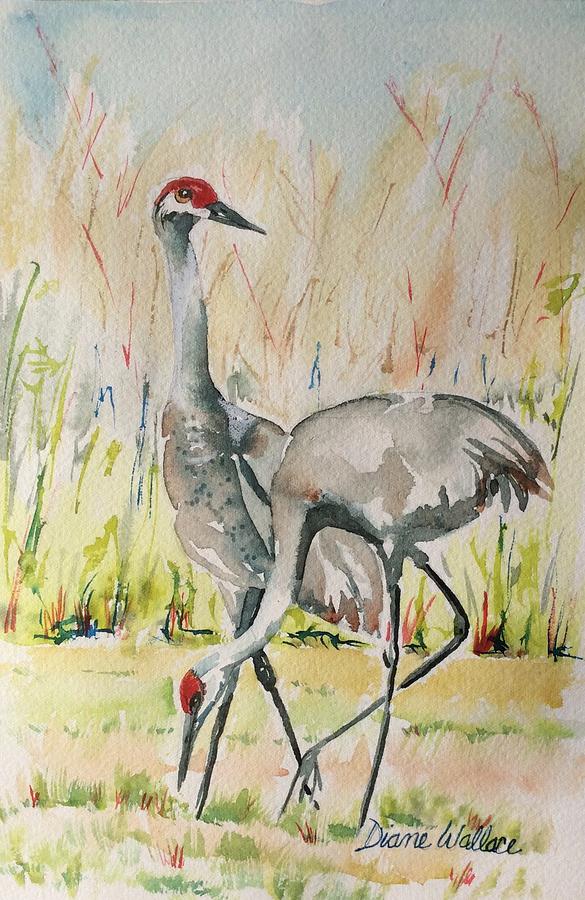The painting depicts two elegant birds, resembling storks or cranes, rendered in delicate watercolor. These grayish birds exhibit distinctive features: they have long necks, black beaks, and bright red patches on the tops of their heads. Both birds possess remarkably long legs. Positioned centrally in the image, one bird, to the left and slightly behind, gazes to the right side of the painting, while the other bird, on the right, bends forward, seemingly engrossed in nibbling on the lush green grass below. The background features a mix of tall green grass transitioning into subdued washes of red and brown, suggestive of a natural terrain. Above, a clear blue sky hints at daytime. In the lower right corner, the artist's signature, "Diane Wallace," is inscribed with a dark blue pen, marking the piece with a personal touch.